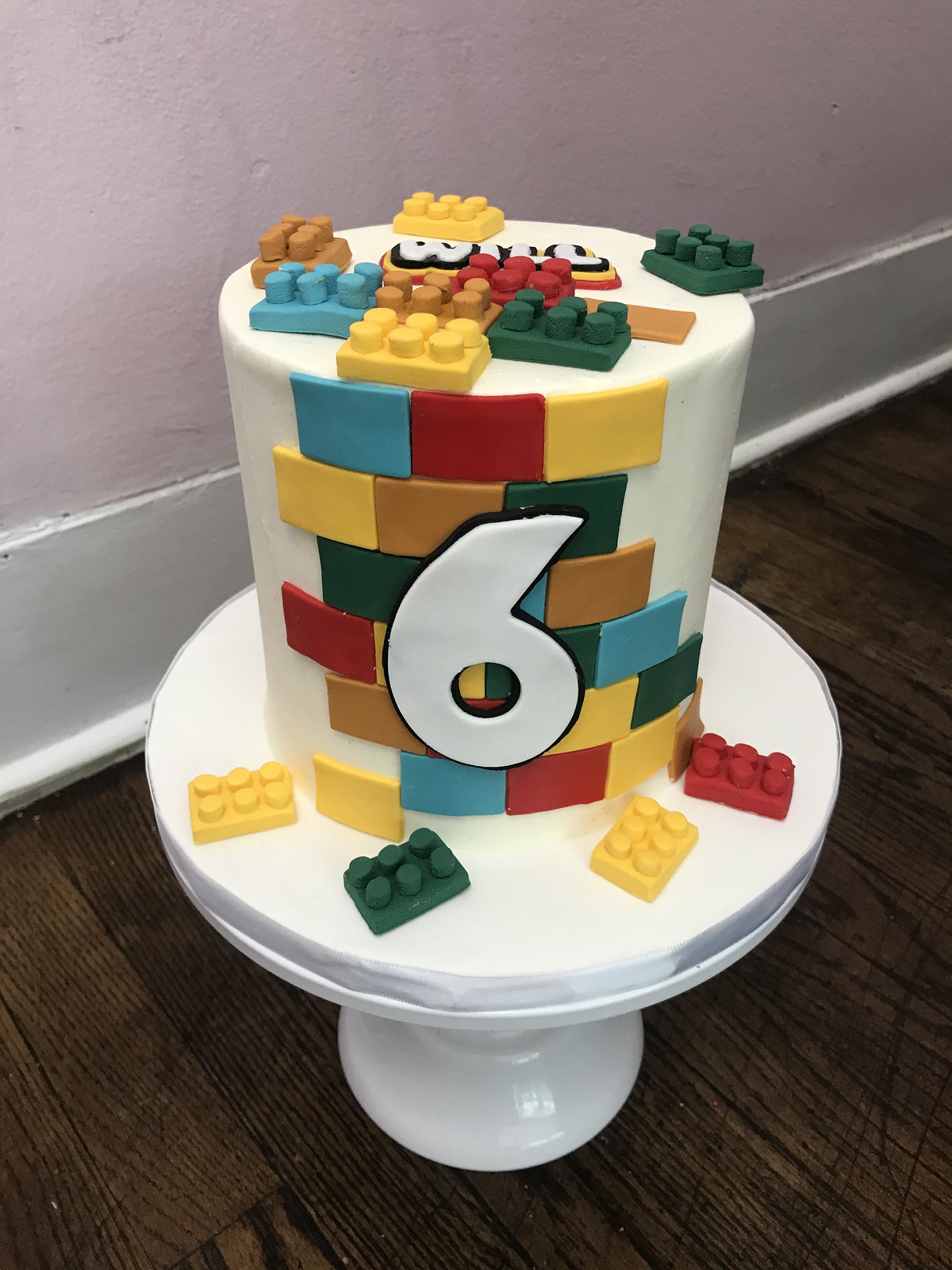The image features a birthday cake designed to resemble a Lego-themed confection. The cake rests on a pristine, white porcelain or plastic cake stand, which is placed on a deep brown, wooden floor with distinct strip lines. The backdrop is a light pink wall with a white baseboard. The cake itself is tall and cylindrical, covered in smooth white frosting. Decorative Lego blocks in vibrant colors of yellow, green, blue, red, brown, and tan adorn the cake. These blocks are arranged in rows around the cake, with additional Lego pieces scattered on the cake stand. A prominent white number "6" is displayed on the side of the cake, possibly bordered in black frosting, signifying a celebration for a six-year-old.